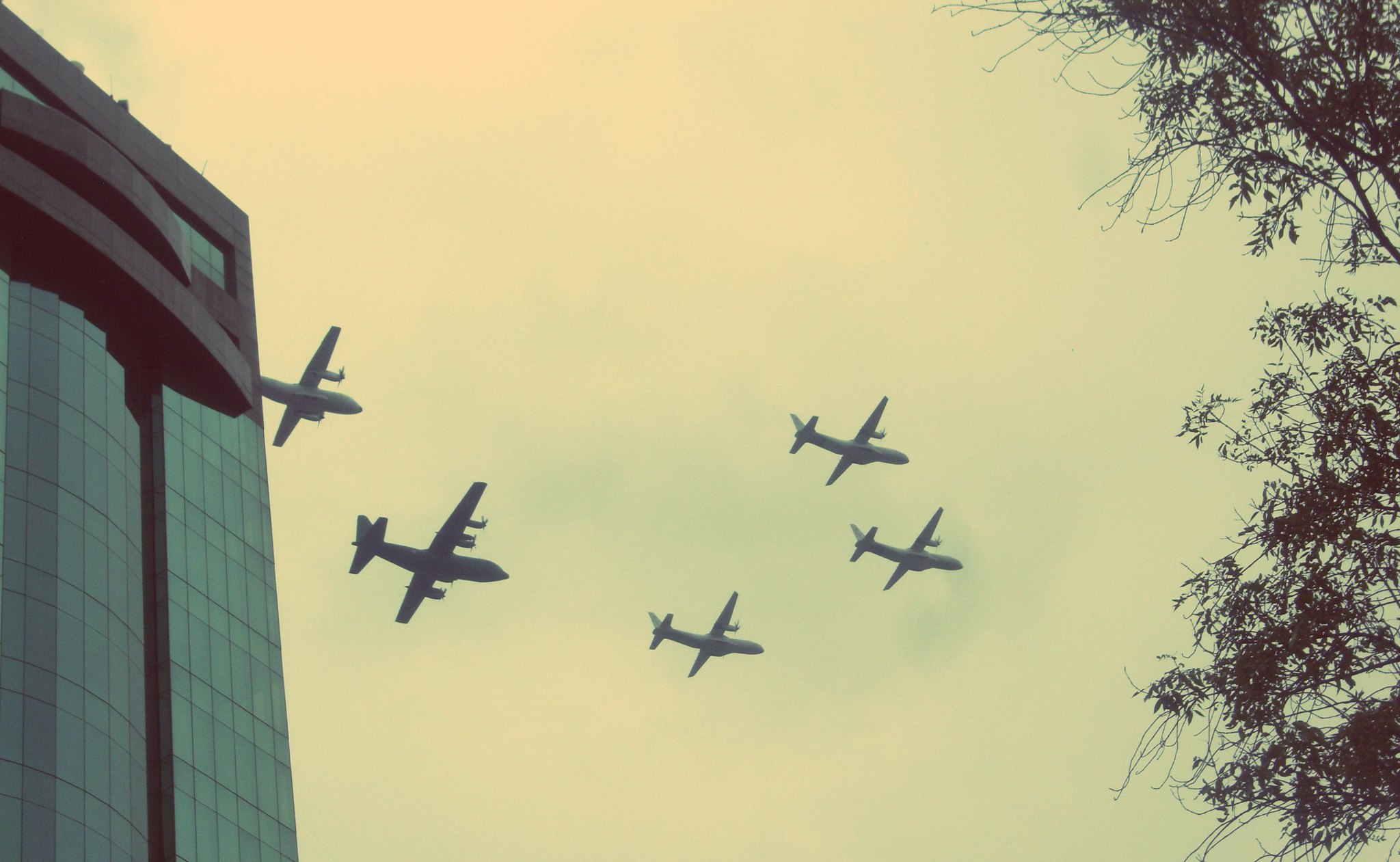This image appears to be an old photograph with a striking yellowish and greenish tint, perhaps indicating a filter or the effect of age on the colors. The picture captures five military airplanes flying through the sky from left to right. On the left side of the image, there is a tall building with a dark facade and bluish windows, possibly an office building or hotel, that spans several stories. On the right side, tree branches with leaves are visible, suggesting the photo was not taken in winter.

The sky has an unusual hazy, almost wildfire-like appearance with orangey-red clouds at the top, contributing to the dated feel of the image. The airplanes are propeller-driven, with varying configurations: four engines are visible on some of the planes. Two larger planes are following three smaller planes, which are flying in a loose V-shape formation. The aircraft are distinctly military in nature, with some planes appearing darker than others due to lighting or their position in the sky.